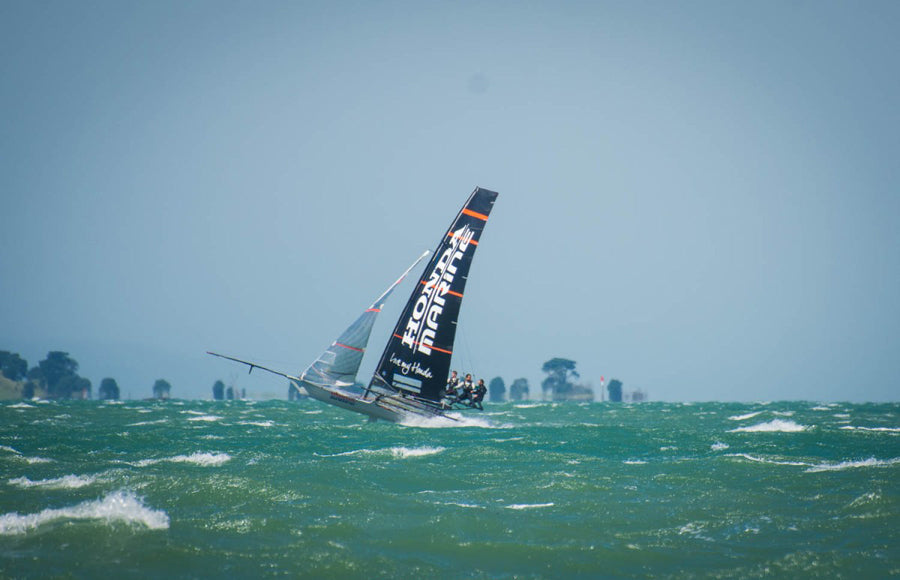The image depicts a sailboat navigating through a tumultuous ocean, with choppy, greenish water marked by white caps. The boat, showcasing two prominent sails—one gray-striped with orange and a larger, navy-blue, striped with orange sail displaying "Honda Marine" in white lettering—has its nose poking out of the water as if it's about to tip over. Three individuals are seen hanging off the side, steering the distressed vessel. The background reveals silhouettes of various trees, possibly palm trees, and an indistinct cityscape under a gloomy, dark sky, adding to the dramatic atmosphere of what appears to be a sports sailing competition captured in a blurry photo.